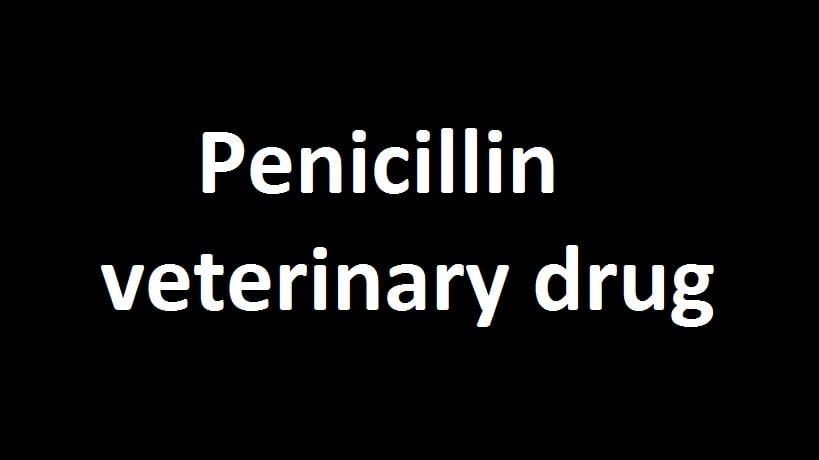The image showcases simplistic white text displayed on a jet-black background. The text reads "Penicillin Veterinary Drug" and is entirely centered. "Penicillin," with the first letter capitalized, occupies its own line and sits slightly off-center towards the left. Below it, "veterinary drug" appears in all lowercase letters, aligning directly underneath "Penicillin." The font used is Calibri, bold, and uniform in size, with no additional shapes, borders, or decorative elements, ensuring the focus remains solely on the text itself.